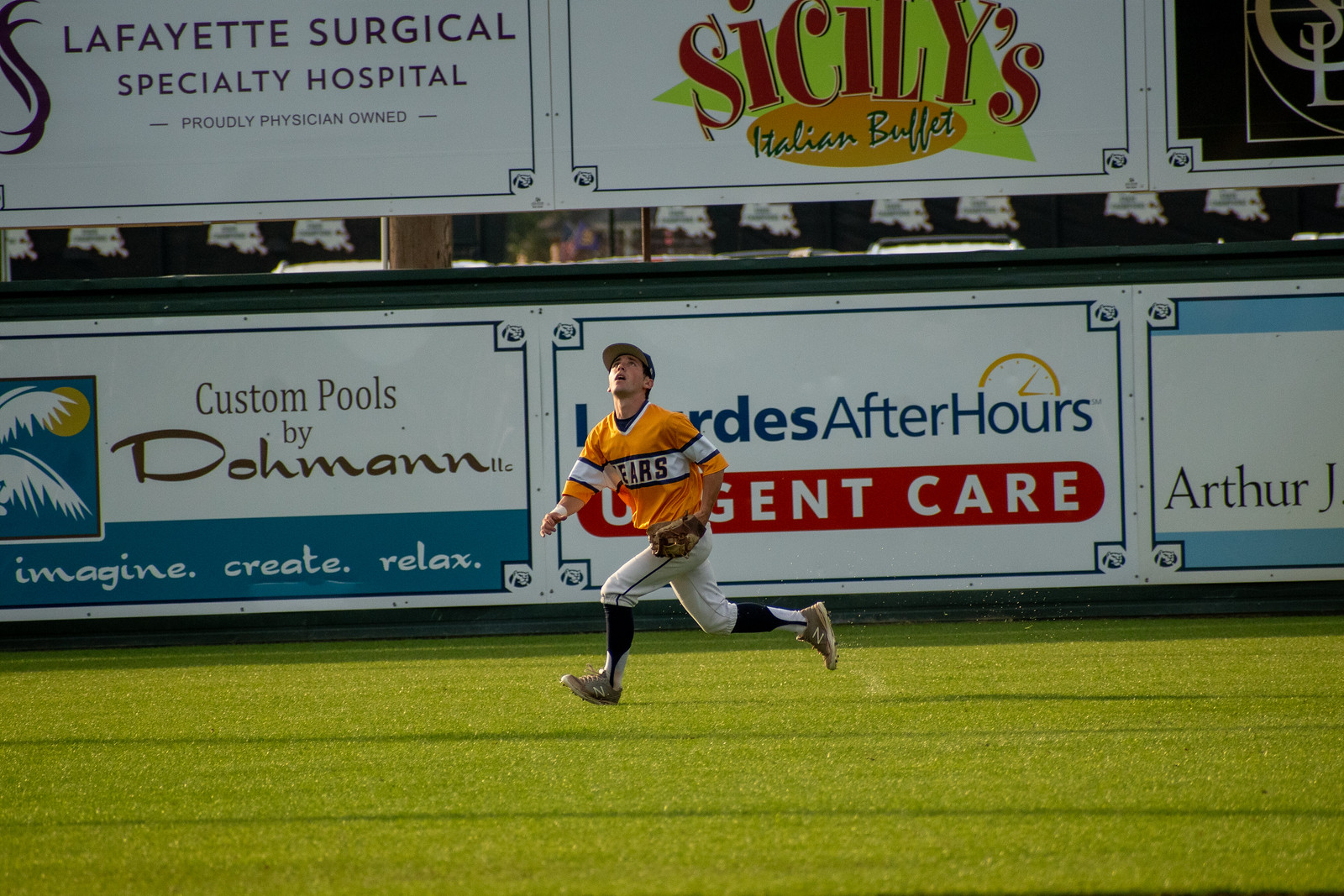In the image, a baseball player is captured mid-run on a grassy field, looking up with concentration as he attempts to catch a ball. He is wearing a light orange jersey featuring white stripes across the body and arms, along with the visible letters "E-A-R-S." Complementing his uniform are white pants, black socks, cleats, and a baseball cap with the bill shading his eyes. The player's left hand sports a glove, while his right hand is outstretched, adding to the dynamic nature of the scene. In the background, several sponsor boards are visible, including signs for Lafayette Surgical Specialty Hospital with the tagline "Proudly Physician Owned," Sicily's Italian Buffet, Custom Pools by Donman with the phrase "Imagine Creates Relax," After Hours Urgent Care, and OrthoJ. The field's green grass and shadows add depth to the composition, highlighting the player's athleticism in this high-stakes moment.